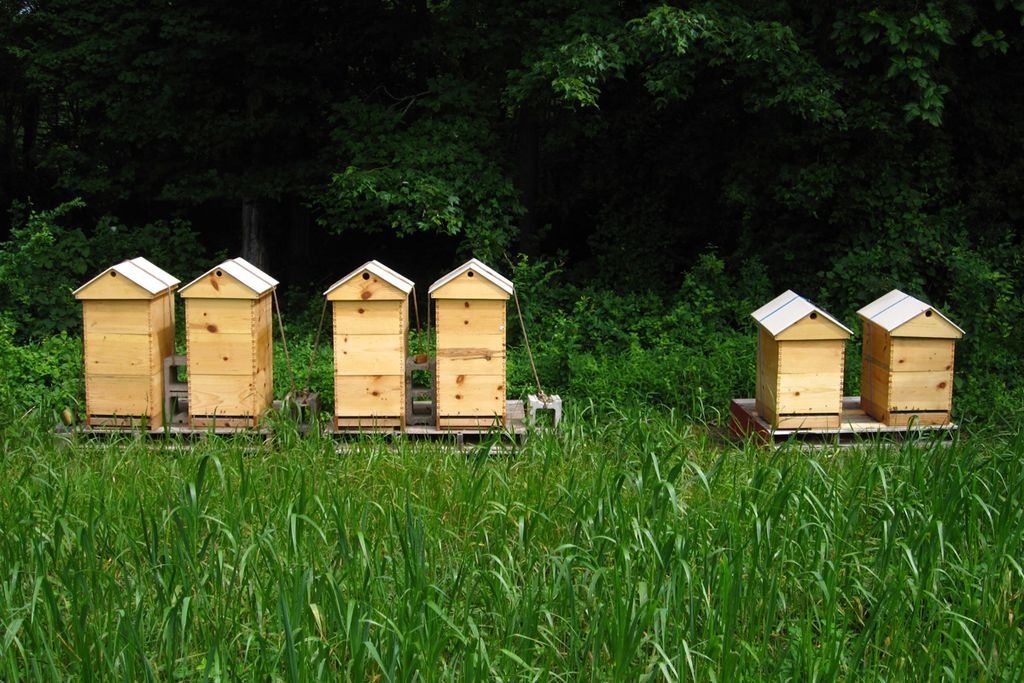In the image, there are six small wooden beehive structures positioned on three wooden pallets in a grassy field. The grass in the foreground is tall and lush, leading up to the beehives, which are placed on the far side of the field. These beehives are crafted from light brown, unpainted wood, and each features a white, triangular gable roof with a rounded entrance hole just below the peak. Stacked in pairs on each pallet, the beehives are arranged with four of them being taller and two, positioned to the right, being slightly shorter. Some of the hives have small cinder blocks next to them with strings extending up to the roofs. In the background, a dense forest with thick foliage obscures the trunks of the trees, adding a rich, green backdrop to the scene.